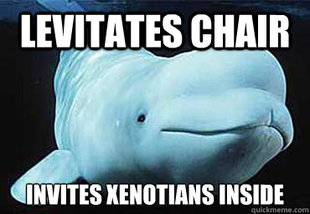In a dimly lit bedroom with dark charcoal grey walls, there's a large bed featuring a dark brown headboard flanked by two bedposts. The bed is adorned with black leather cushions with white stripes, black sheets, and a multicolored comforter with red, white, black, and gray patterns. In the center of the bed, a muscular, bald man with a beard, goatee, and a tattoo on his right shoulder is positioned on all fours. Wearing only underwear and looking directly at the camera with a hint of guilt or humor, he has a black cylindrical object with white stripes placed beneath his abdomen. Below him, in bold white text with a black border, the word "HAI" is prominently displayed. The surrounding space includes details like white electrical outlets on the walls beside the bed.